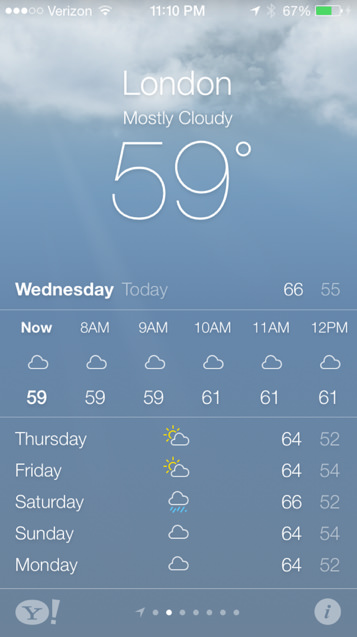The image depicts a weather application displayed on an iPhone. At the top of the screen, the status bar shows "Verizon" as the carrier, the time as "11:10 PM," and a battery level at 67%, indicated by a green battery icon. 

The background features a serene blue sky adorned with light, fluffy white clouds along the top edge. Central to the screen is the weather information for London, which is described as "mostly cloudy" with a current temperature of 59°F, displayed prominently in large letters.

Below, the app details the day's forecast: 

- Wednesday: 
  - Today's range: 65°F (high) and 55°F (low).
  - Hourly forecast from 8 AM to 12 PM: steady at 59°F until 11 AM, then increases to 61°F. Cloud icons are shown for each hour.

Further down, the extended forecast lists the weather for the upcoming days:

- Thursday: 64°F / 52°F - Partly Cloudy
- Friday: 64°F / 54°F - Partly Cloudy
- Saturday: 66°F / 52°F - Rainy
- Sunday: 66°F / 54°F - Cloudy
- Monday: 64°F / 52°F - Cloudy

In the lower-left corner, there is the Yahoo Weather logo, featuring a "Y" with an exclamation point. An information icon is present nearby. 

At the bottom, there is a horizontal scroll menu with various icons representing different sections or saved cities, with the second icon currently selected. Only the weather information for London is visible on this screen. 

Finally, the upper-left corner of the screen shows the Verizon logo once more, affirming the carrier.